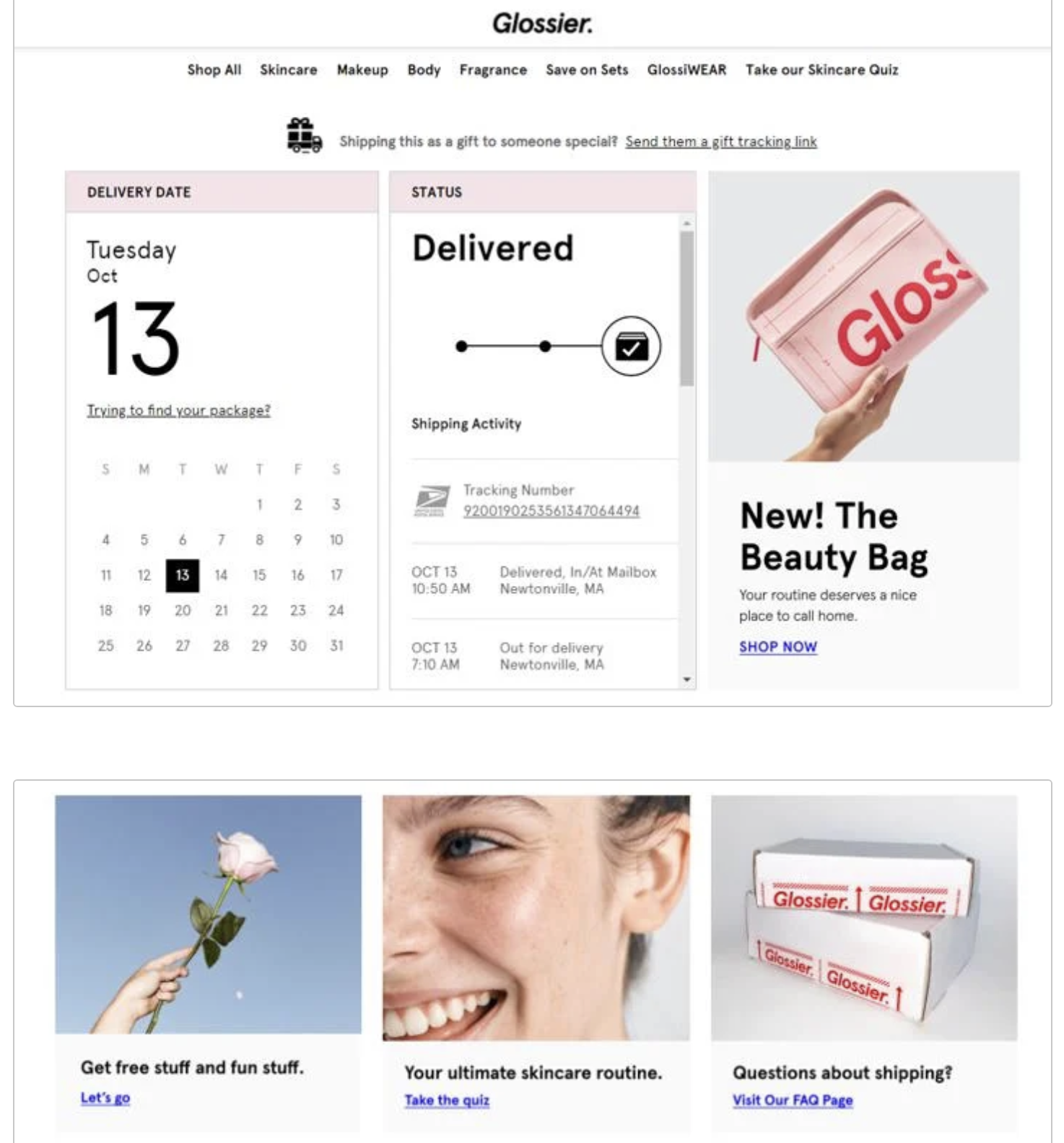This image is a detailed screenshot of a Glossier web page, featuring a white background. At the top of the page, "glossier." is clearly written in black text, followed by a horizontal menu bar containing various black menu items: Shop All, Skincare, Makeup, Body Fragrance, Save on Sets, GlossiWEAR, and Take Our Skincare Quiz.

Beneath the menu, there's a logo of a truck with a large present on its back, accompanied by the text: "Shipping this as a gift to someone special? Send them a gift tracking link."

On the left side of the page, there's a prominent pink date, "Tuesday, October 13th," indicating the delivery date. This section also includes a prompt: "Trying to find your package?" accompanied by an image of a calendar with "Tuesday the 13th" highlighted in a black box.

To the right, a pink box announces the "Status: Delivered," providing detailed shipping activity. It shows the tracking number and indicates that the package was delivered to a mailbox in Newtonville, Massachusetts, at 10:50 a.m. on October 13th and was last out for delivery at 7:10 a.m. the same day.

On the right-hand side, there is an advertisement featuring a gray square with a person's hand holding a pink bag labeled "gloss" in red text. Below this image, bold black text proclaims "NEW: The Beauty Bag," accompanied by the tagline, "Your routine deserves a nice place to call home," and a blue clickable link that says "Shop Now."